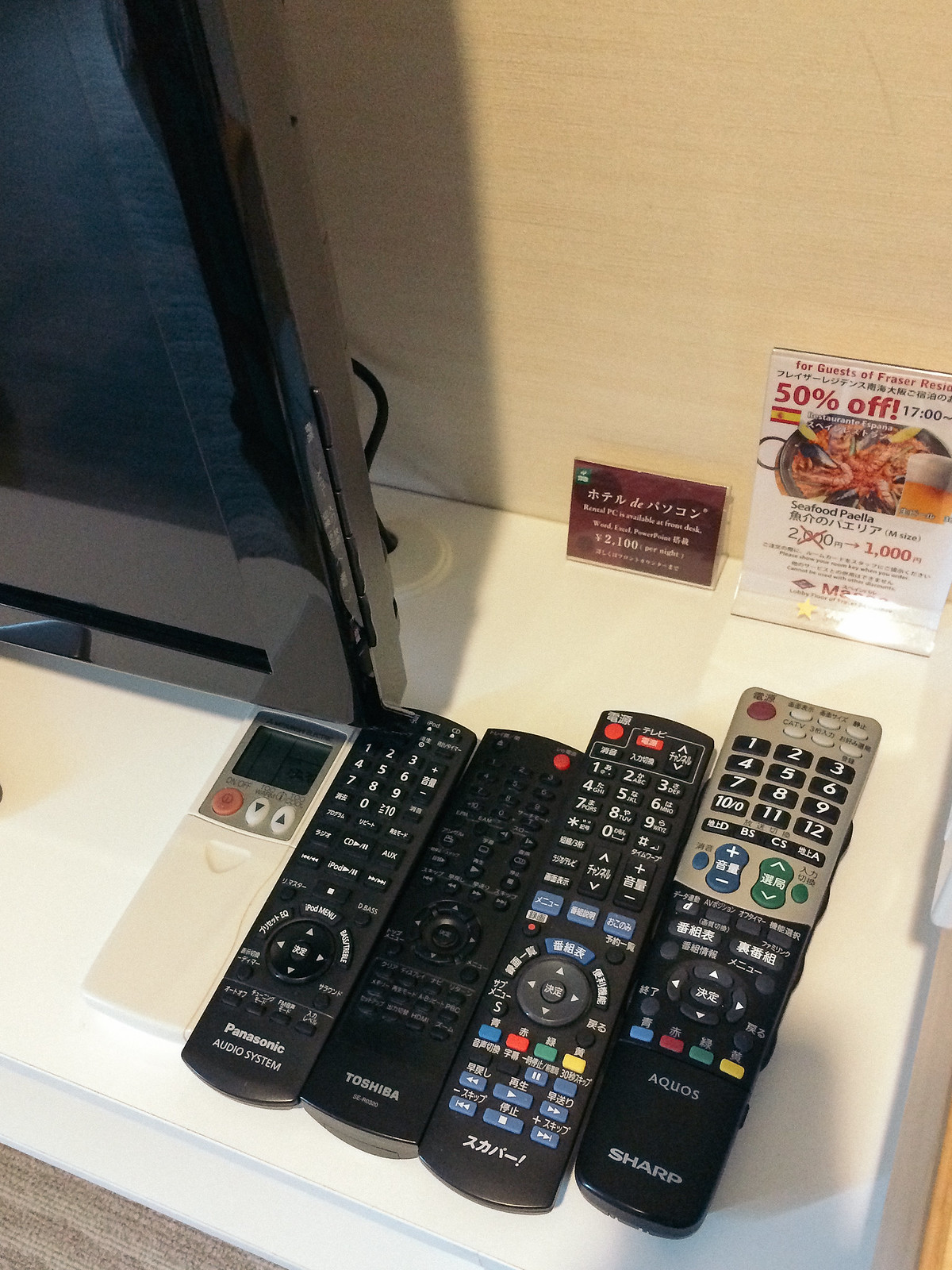This photograph captures a scene inside a bedroom featuring a white desk or stand positioned against a tannish-white wall. Resting on the desk's smooth, flat surface are five TV remotes arranged in a line from left to right, progressing from shortest to tallest. At the far left is a white remote, followed by three black remotes, and at the far right, a black and silver remote. Brands identified include Panasonic, Toshiba, and Sharp, with some remotes labeled in an Eastern Asian language.

In the upper left of the image, the edge of a black television or monitor screen is visible. The upper area of the desk also holds two small advertisements. The larger sign is white and promotes a seafood paella dish with a special offer, and the smaller sign, with a red background and white foreign text, displays the number 2100. Additional details include a glimpse of a beige carpet on the floor.